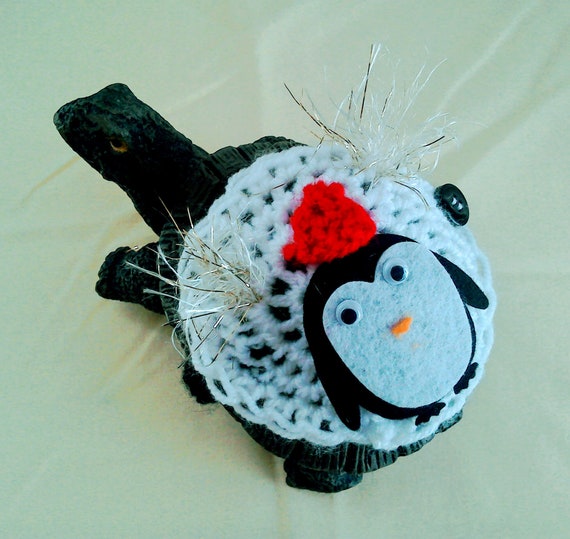The image captures a whimsical arts and crafts scene featuring a crochet turtle resting on a light green, seafoam-colored background. The turtle, crafted in dark green yarn with gleaming yellow eyes, sports a light blue crocheted shell adorned with sparkly tinsel. Perched atop the shell is a playful penguin fabric design. The penguin, characterized by its black body and sky blue face, has googly eyes and a small orange beak. It wears a red crocheted patch resembling a hat and features additional black flippers and feet. Overall, this endearing combination showcases a creatively layered handmade project with attention to detail and a charming mix of colors and textures.